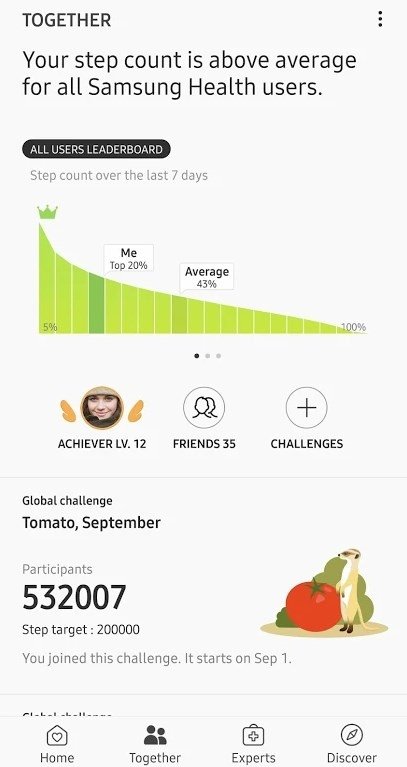The image displays a detailed dashboard from the Samsung Health app, highlighting various fitness statistics and community challenges. At the top, the average step count for the last 7 days is shown, indicating that the user's step count is above average compared to all Samsung Health users. The user ranks in the top 20% on the global leaderboard, where the average user ranks at 43%. The user's achiever level is 12, and they have 35 friends connected through the app.

Additionally, information about ongoing challenges is visible. One highlighted challenge is the "Global Challenge" led by Sumitra for the month of September, with 532,007 participants and a target of 200,000 steps. The image notes that the user has joined this challenge, which starts on September 1st. 

The dashboard is organized into various categories for easy navigation: "At Home," "Together," "Experts," and "Discover," providing users with tailored content and community support.